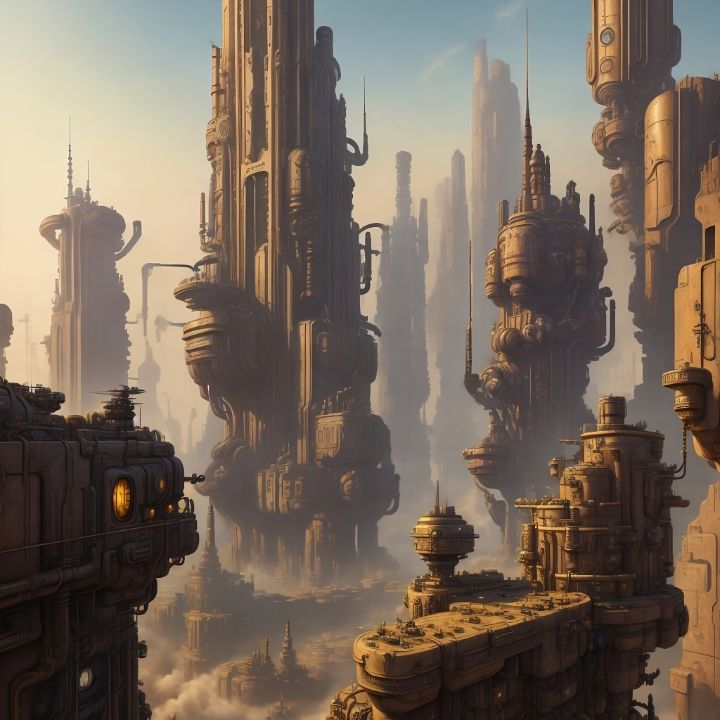This image is an artistic rendition of a futuristic, possibly cyberpunk or steampunk, cityscape set in a dusty or smoggy environment, which might be a desert or a barren planet. The scene is dominated by a myriad of towering, cylindrical buildings with phallic-like shapes, giving it an industrial and mechanical feel. These structures, mostly bronze or brown in color, vary greatly in design, featuring spires, bulbous extensions, and various appendages like platforms and handles. Many buildings have glowing windows or illuminated sections casting a yellow or orange light, particularly noticeable in the darker foreground where a round, brightly lit window is present, possibly part of a domed or submarine-like structure. The base of the city is enveloped in a thick haze, through which only the top parts of the buildings and a small patch of blue sky in the upper right corner are visible. The cityscape lacks any signs of vegetation, life, or greenery, enhancing its desolate and industrial atmosphere. The overall aesthetic is mid-century modern with muted colors, metallic textures, and an arrangement that hints at a chaotic yet meticulously constructed urban jungle.